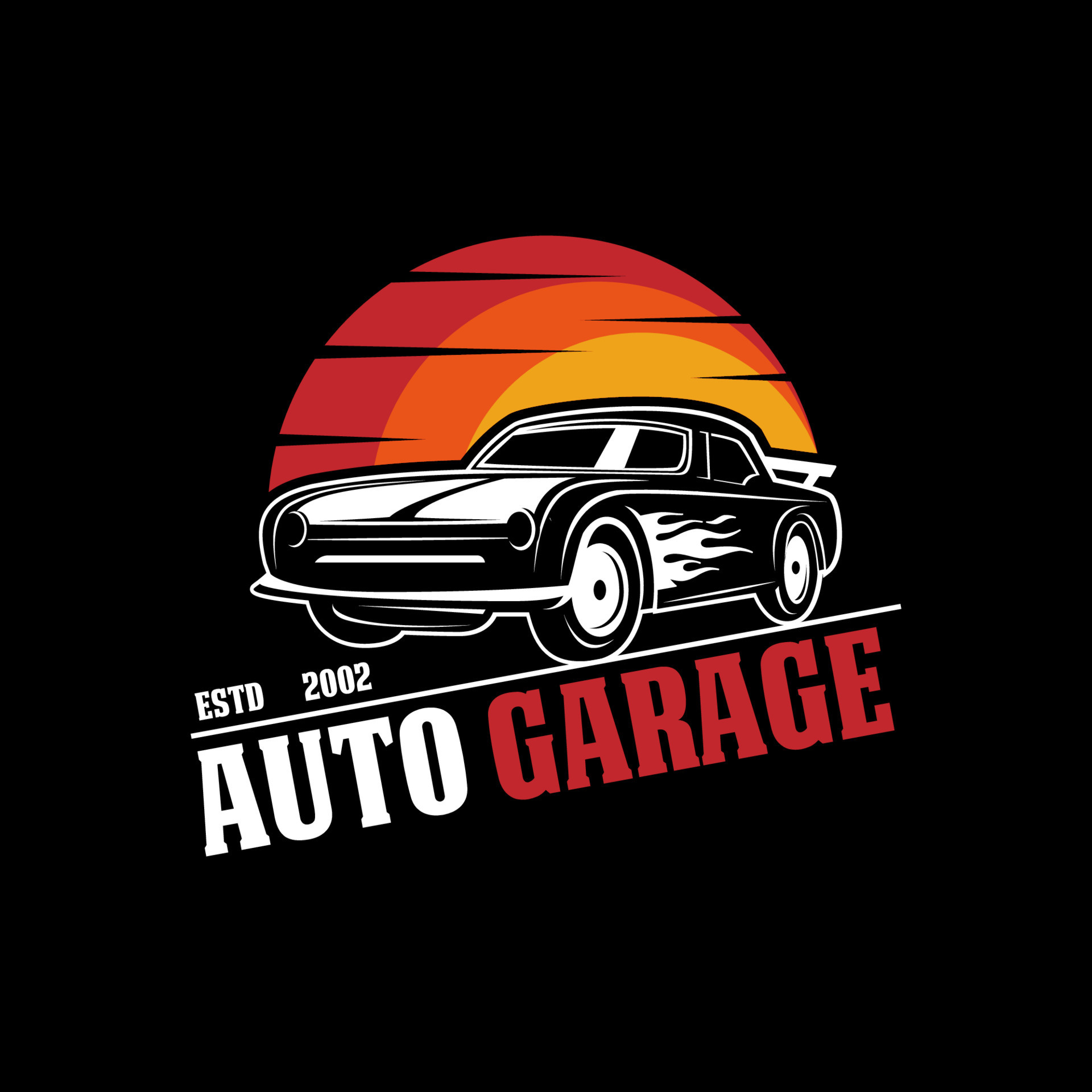The image is a logo with a black background featuring a central design. At the top is a sunset art print, resembling a logo or sticker, with three partial circles in dark yellow, orange, and red tones, each with thin black horizontal stripes. Below the sunset, there's a black and white clip art of a sports car, facing left, adorned with white flames on its side and a prominent tail fin. The car appears to be speeding, emphasizing its dynamic look. Centered beneath the car's wheels is the text "ESTD 2002" in white, followed by a horizontal white line. Below this line are the words "AUTO" in white and "GARAGE" in red, both in all uppercase letters. The text is slightly angled, adding to the sense of motion and energy conveyed by the car.